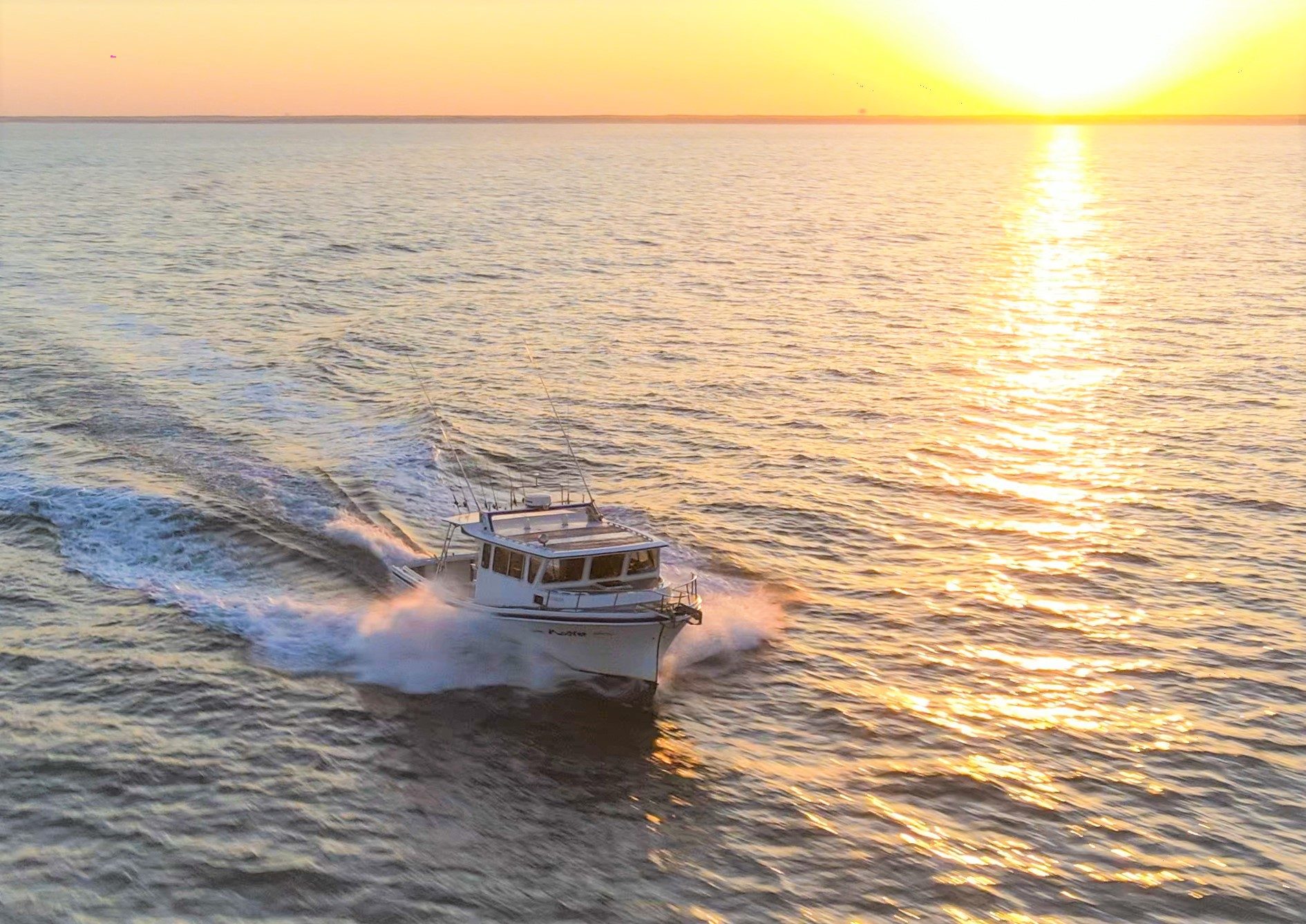This photograph captures a dynamic scene of a white and blue-trimmed fishing boat speeding through a vast body of water, either a lake or the ocean, with splashes cascading off both sides. The boat is sizable, estimated at 18-20 feet, and equipped with a captain's deck and various antennas and fishing riggings extending from the roof. The serene background features a sun just at the horizon, painting the sky in brilliant shades of orange and gold, with golden beams reflecting majestically on the water's surface. The water is mostly calm, though slightly choppy near the boat, emphasizing the boat's rapid pace as it creates a notable wake and leaves a streak of illuminated splashes in pastel purples and reflections of the setting or rising sun. The expansive, calm water and the serene golden sky contribute to an overall picturesque and tranquil backdrop, highlighting the stark contrast of the boat’s energetic movement.